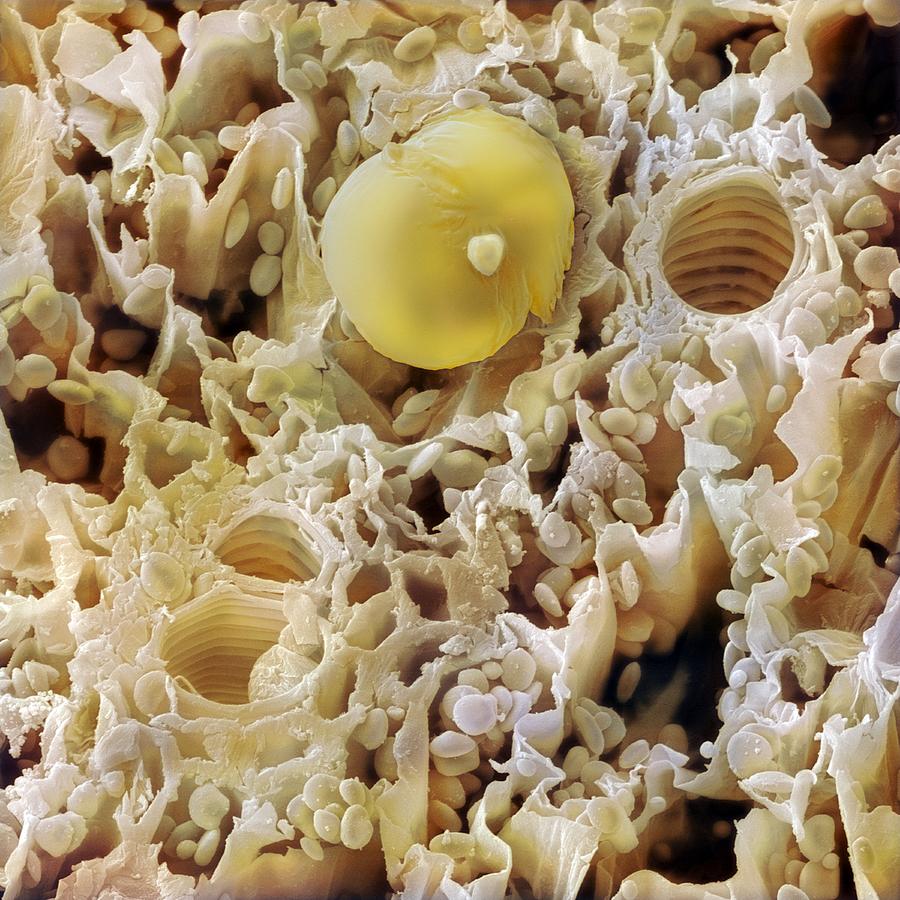This magnified color photograph presents an intricate, organic scene filled with various shapes and sizes of holes, circular objects, and granule-like textures. Dominating the view are hues of white, beige, brown, and yellow, seamlessly blending into an almost abstract composition that spans the entire frame. The image predominantly features an array of organic curves and smooth surfaces, dotted throughout with pebble-like elements reminiscent of tiny river rocks or sesame seeds. At the top center, a prominent, balloon-like structure stands out due to its distinctive yellow shade and a small white dot at its core, drawing the eye in a setting otherwise dominated by ivory and pink tones. The background is a chaotic, non-uniform pattern, somewhat suggesting the texture of a sponge or honeycomb, further enhanced by clusters of the granule-like objects and sporadic dark patches peeking through sparse areas.